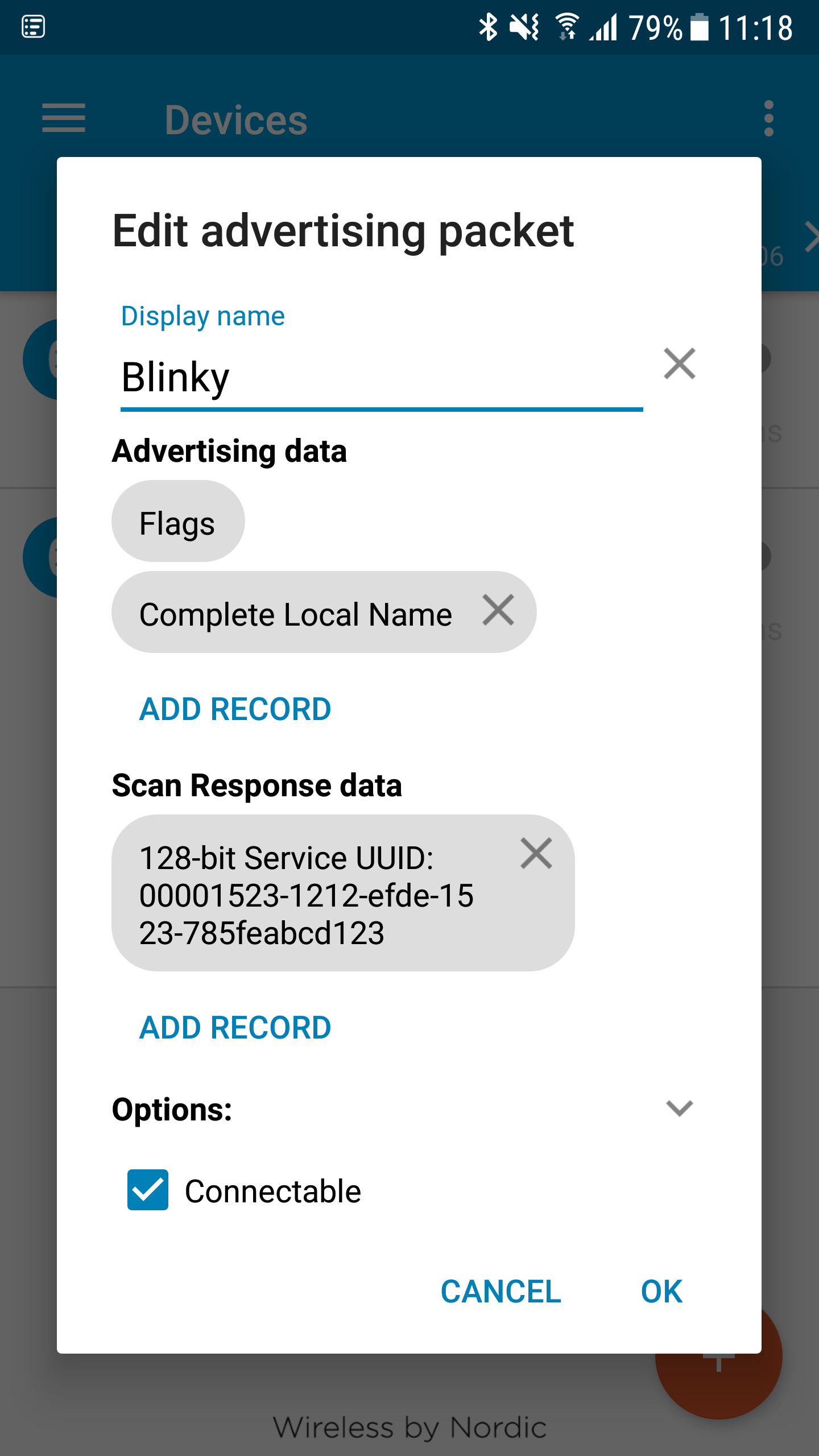**Detailed Caption:**

The image features a pop-up menu overlay against a main background page. The pop-up menu has a clean white background with black text for the majority of its content, except for certain elements that are highlighted in blue. 

At the top, the menu headings include "Advertising Packet" and "Display Name." Beneath these headings, the name "Blinky" is displayed. This is followed by a section labeled "Advertising Data," which contains two selected flags: "Complete Local Name."

Further down, there is a text box labeled "Scan Response Data." Within this box, there is a 128-bit service UUID accompanied by a series of hexadecimal numbers. Beneath this, the option to "Add Record" is also mentioned.

Additionally, there is an "Option" label followed by "Connectable," which has an adjacent checkbox that is checked and blue in color.

At the bottom-right corner of the pop-up, there are two buttons labeled "Cancel" and "Okay," both written in blue text.

In the background of the image, the upper portion of the main page is visible, with a blue background and the word "Devices" written in white. The white pop-up overlay stands out prominently against this blue background. Some elements of the overlay text are also highlighted in blue, such as "Display Name" and "Add Record."

Lastly, at the bottom-right corner of the entire image, there is an orange pattern and the text "Wireless by Nordic." This background detail seems to add a finishing touch to the interface's visual design.